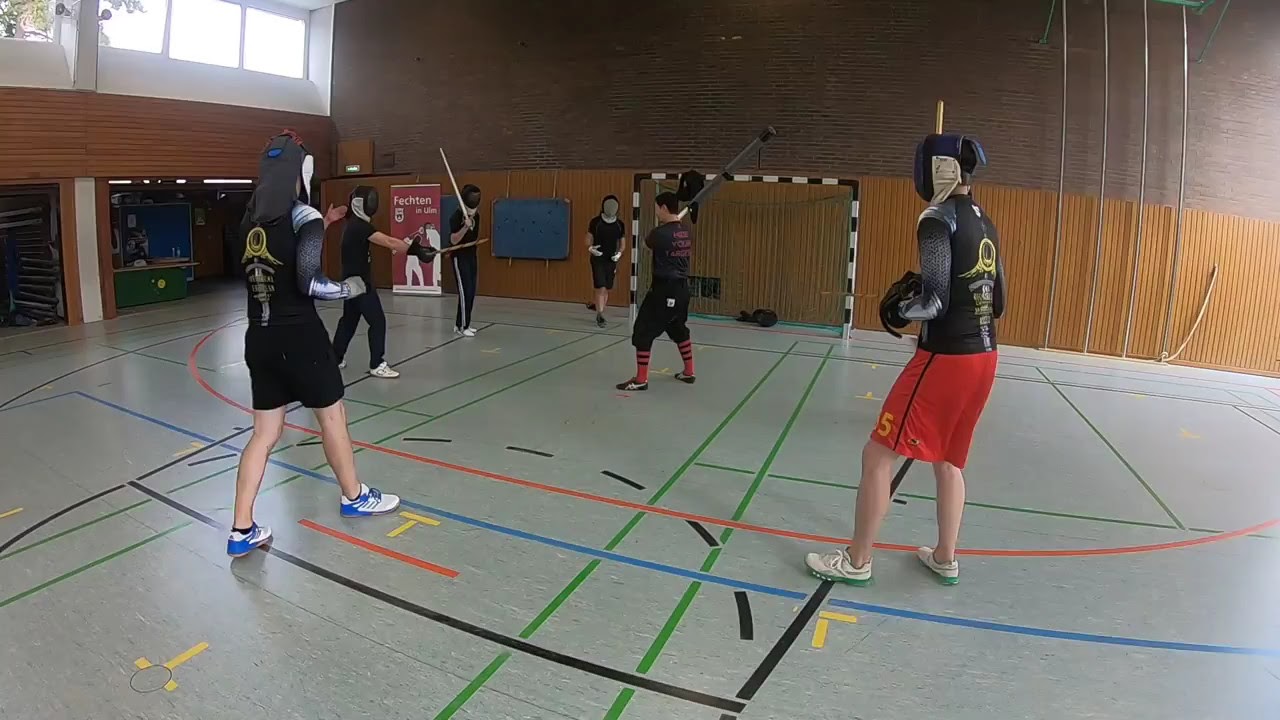The image depicts an indoor kendo training session in what appears to be a multipurpose gymnasium, evidenced by the various colored lines delineating a basketball court and a soccer goal in the background. There are six participants in total, five of whom are encircling a central figure who is likely the teacher. All participants, except the central figure, are wearing protective headgear and wielding wooden practice swords.

The central figure, identifiable as the teacher, is holding his protective gear in his right hand and appears to be in mid-instruction, directing his attention toward three individuals positioned on the left. He is dressed in black shorts, black shoes, and red socks. The participants' attire consists of standard athletic gear: black shirts, with one individual in a long-sleeve black shirt adorned with a circular emblem resembling two points and a spine or hatchet. The participants' lower attire varies from black pants, some with white stripes, to shorts.

One of the tallest individuals, positioned to the right of the central figure, is distinctly attired in a red shirt, black protective gear, and white shoes. This individual appears muscular, with protective mitts visible on his left hand. The scene is set against a backdrop of wood-paneled walls, exposed piping, and a window situated in the top left of the image, suggesting the gym's multifunctional use and utilitarian design.